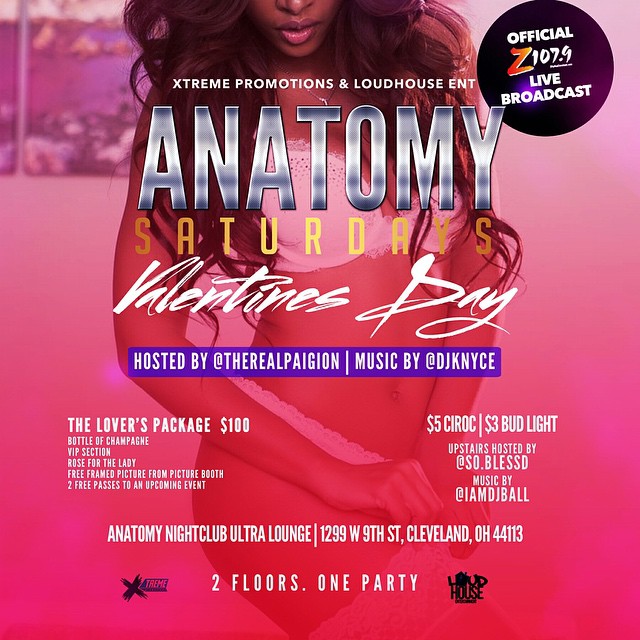The advertisement poster features a striking red background with a central image of a woman cut off at the nose, her long black hair cascading down as she poses in pink lingerie, slightly turning her lower body to the right. She has her right arm down along her body and her left arm at her waist. 

Across the top, in small white letters, it reads “Extreme Promotions and Loud House Entertainment,” just below her chin. Below, large silver letters spell out “Anatomy,” followed by “Saturdays” in bold yellow and “Valentine's Day” in cursive white. 

The flyer includes various details such as “Hosted by The Real Pagan” and “Music by DJ Nice.” Additional information is presented in blue boxes, including a “Lover’s Package” for $100, which offers a bottle of champagne, VIP section, rose for the lady, free framed picture, and two free passes to an upcoming event. 

On the left side of the image, it mentions $5 Ciroc and $3 Bud Light. The name "Anatomy Club Ultra Lounge" and its address, 1299 West Ninth Street, Cleveland, Ohio, are prominently displayed at the bottom. Below that, it states, “Two floors, one party” in white, flanked by emblems on each side. The upper right corner features a black circle with the words “Official Z 107.9 Live Broadcast.”

Overall, this flyer is designed as an eye-catching promotion for a nightclub event, emphasizing vibrant colors, enticing offers, and detailed event information.